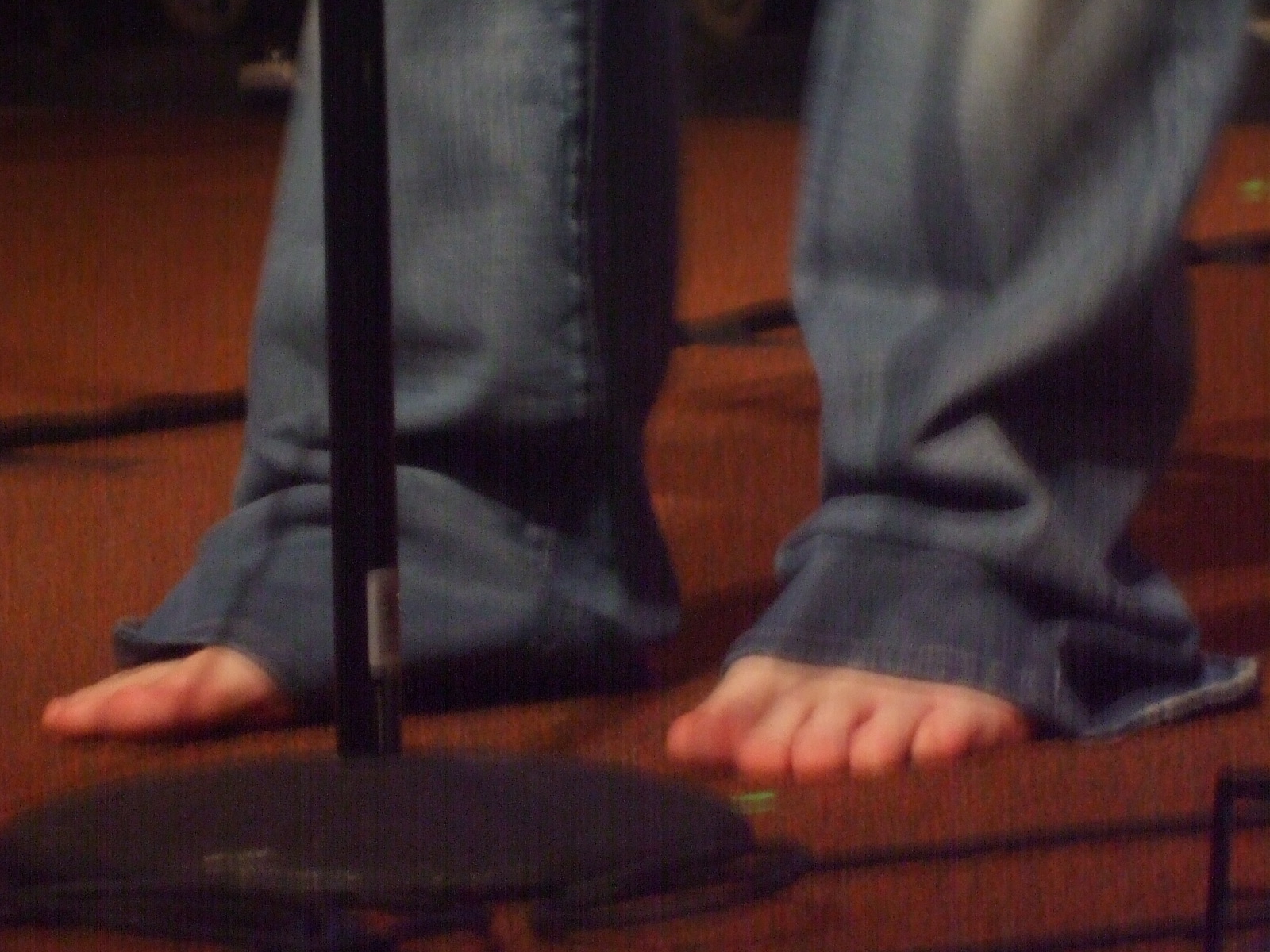The photograph showcases a horizontally oriented rectangular image, primarily focusing on a person standing on a stage. The individual is adorned in oversized, dark blue jeans that extend all the way to the floor, concealing most of their legs and revealing only their bare toes. The excess length of the jeans causes them to bunch up and drag on the stage, creating a casual yet striking visual.

In the lower left corner of the image, the round base of a microphone stand is visible, with a black pole rising from it. A microphone cord snakes across the right side of the stage, meandering off-frame. The stage floor itself is predominantly a brown or orange hue, with a distinct black stripe cutting across the middle of the image, providing contrast to the scene.

The person’s legs dominate the center of the photograph, with the perspective cutting off just below the knees, emphasizing the oversized nature of their attire and the grounded, barefooted stance they have adopted on this warmly lit stage.